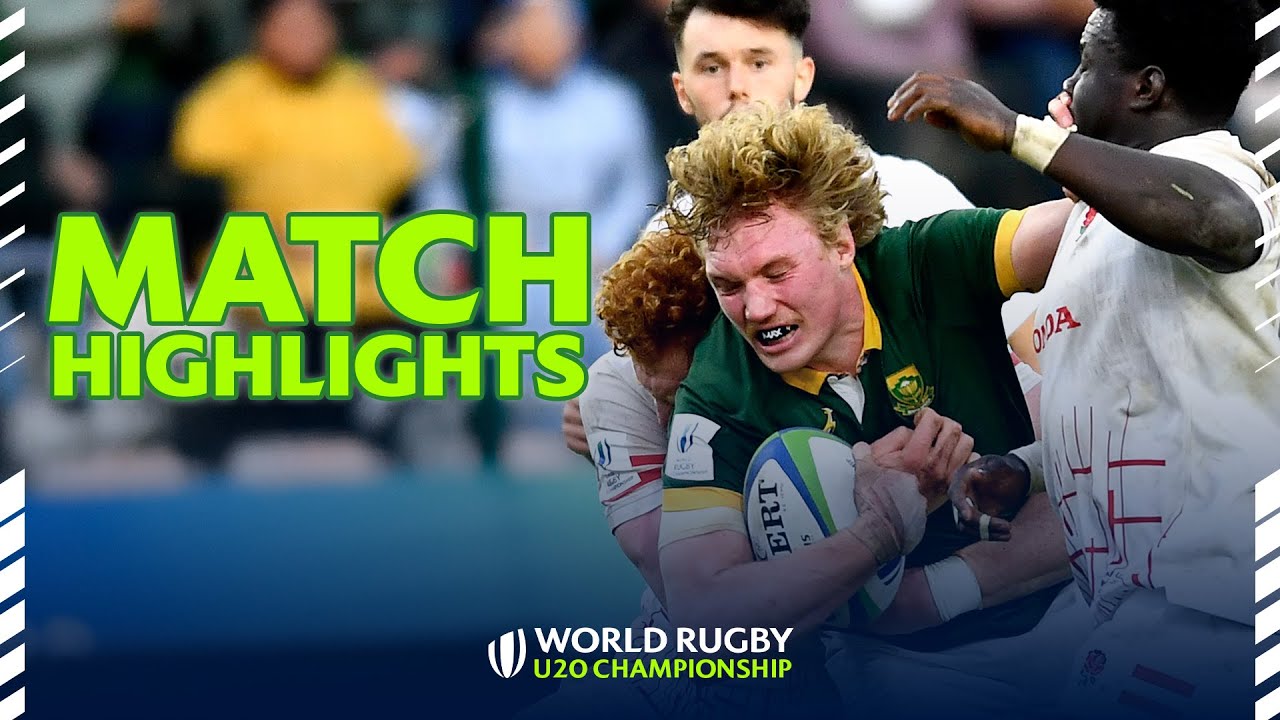In this dynamic image capturing a moment from the World Rugby U-20 Championship, the focal point is a robust match highlight scene. Dominating the left side in bright green capital letters, edged in darker green, is the text "MATCH HIGHLIGHTS." Below, the event title "World Rugby U-20 Championship" is prominently displayed. The right-hand side of the photo showcases the intense action: a Caucasian player with flowing reddish blonde hair, wearing a green shirt trimmed in yellow with a white undershirt, clutches a rugby ball under his arm, his other hand raised against the face of an opponent. This opponent, a black man in a white shirt with red stencil designs, is close by, seemingly struggling to grapple him. Another player in a white shirt with red stripes is positioned close to the ball carrier's shoulder. A third figure, blurred in the background, watches the scene unfold, adding depth to the competitive atmosphere. The image captures the raw physicality and strategic maneuvers characteristic of rugby.